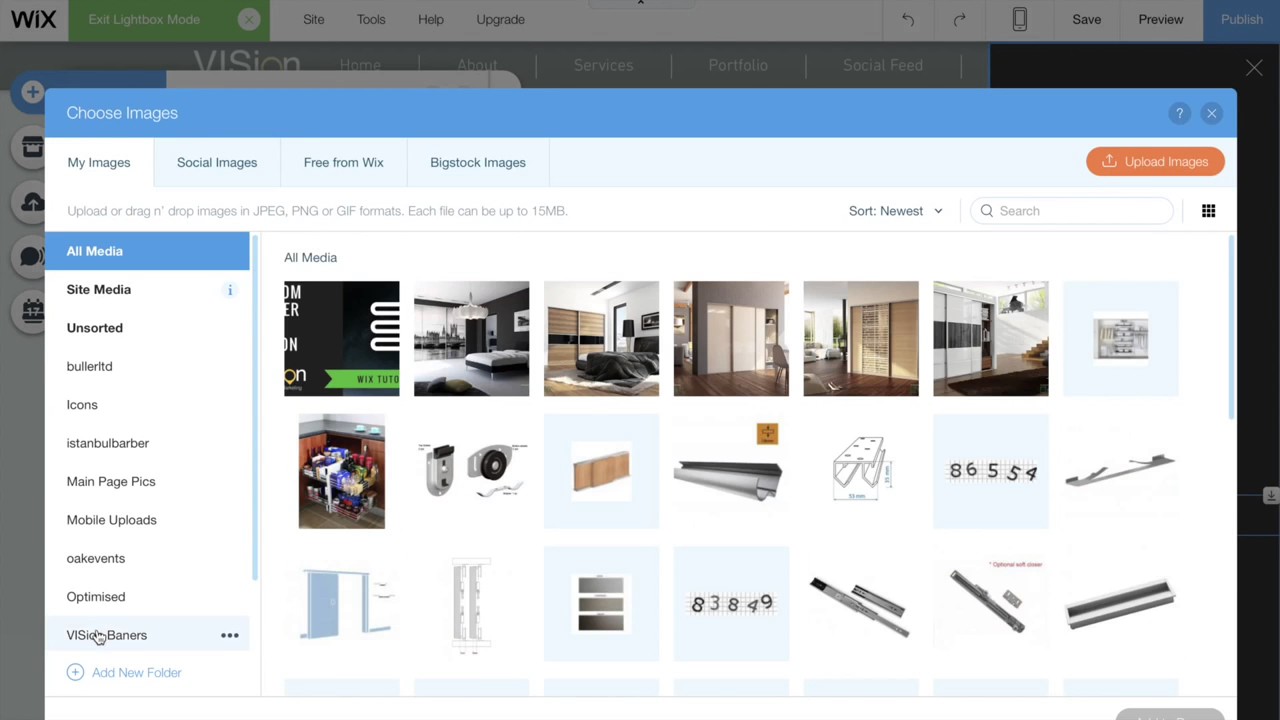The image is a screenshot from a website, illustrating a user interface for selecting and uploading images. The top of the website is slightly darkened due to an active pop-up, which stands out with a blue banner labeled "Choose Images." Below, within a white background, there are clickable options labeled "My Images," "Social Images," "Free from Wix," and "Stock Images."

On the right side of the pop-up, an orange banner with an upward arrow bears the text "Upload Images." Below it, there is an instructional text stating, "Upload or drag and drop images in JPEG, PNG, or GIF formats. Each file can be up to 15 MB."

The left-side menu displays a list of media categories. The first item, "All Media," is highlighted in blue with white text. The subsequent items are in black text, including "Site Media," "Unsorted," "Booler LTD," "Icons," "Instant Bulbarber," "Main Page Pics," "Mobile Uploads," "Oak Events," "Optimized," and partially obscured by a small hand icon, "VIS." The menu also contains "Banners" spelled as "B-A-N-E-R-S."

The main section labelled "All Media" displays various images of rooms and products, offering visual content options for selection or upload.